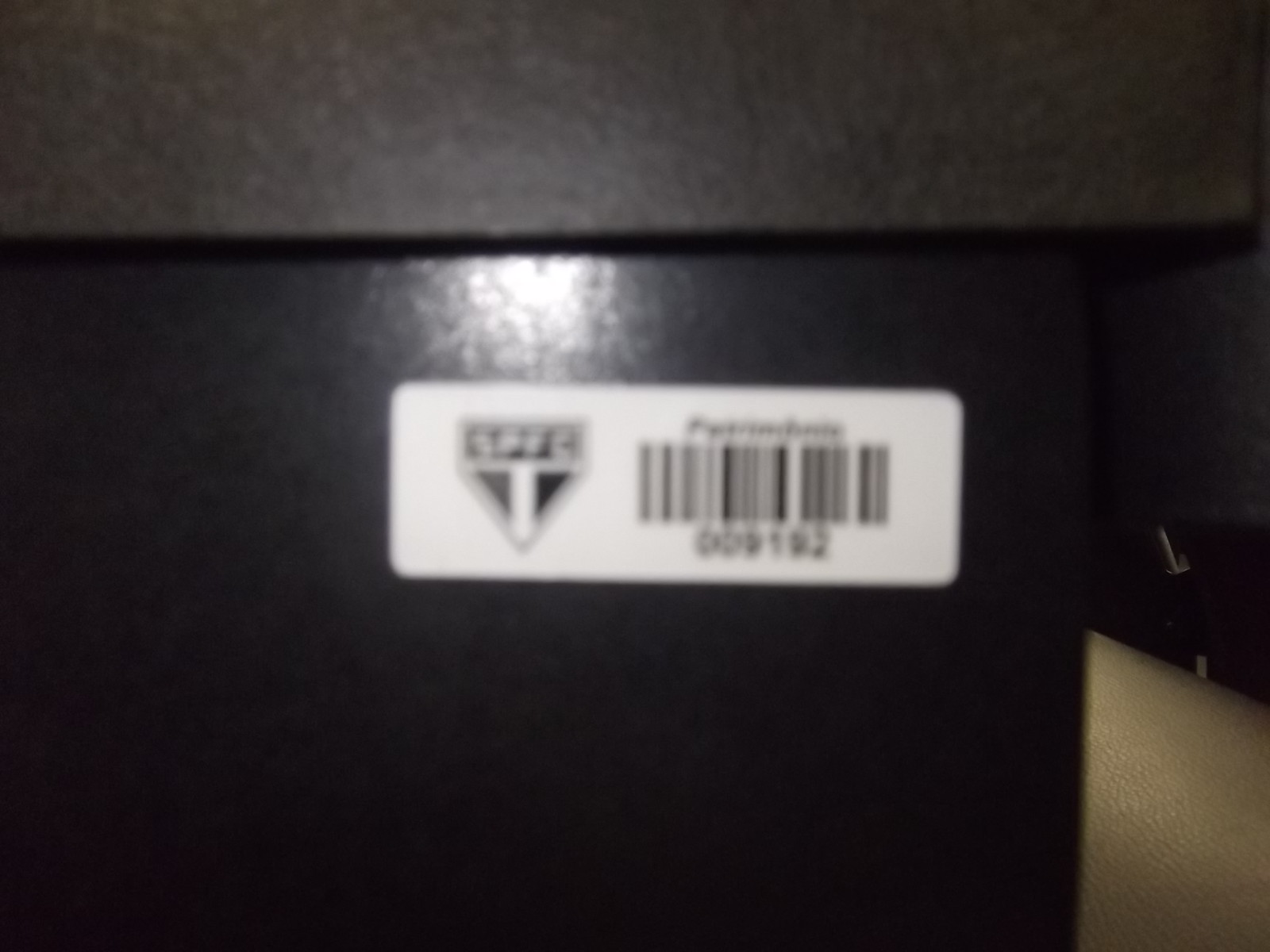This is an out-of-focus, blurry photograph taken with flash, which reflects off the upper center of the image, creating a circle. The image centers on a white label with a black barcode positioned on the right side. This label, found on the back of an electrical or general appliance, also contains some illegible text above the barcode and numbers below it. To the left of the label, there's a home plate-shaped logo containing letters and a partial 'T.' Beside this logo, there is what appears to be a scanner code. The appliance seems to be a black box with a lid that appears slightly too large, dotted with some texture. A tan leather object is visible on the far right, and a light gray piece with another black box above it is also present in the right-hand portion of the image.